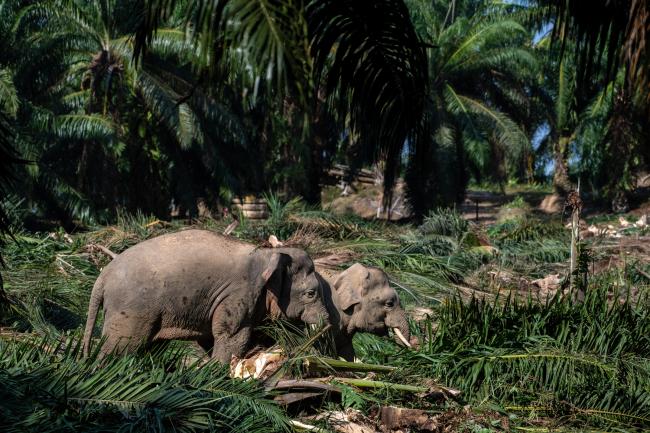In this vibrant outdoor photograph taken in a jungle, two young, dark gray elephants are at the center of the scene, walking through a clearing abundant with cut palm branches and foliage. One elephant stands slightly ahead, obscuring part of the second, but its head and single white tusk are still visible. The elephants' profile captures their calm demeanor as they face right, with their surroundings bathed in lush greenery. In the background, tall palm trees with wide trunks and sprawling, low-hanging fronds stretch towards a patch of blue sky that peeks through the dense canopy, adding depth to this tranquil nature setting. No text intrudes on the image, allowing the viewer to focus solely on the serene companionship of the two elephants amidst their natural habitat.